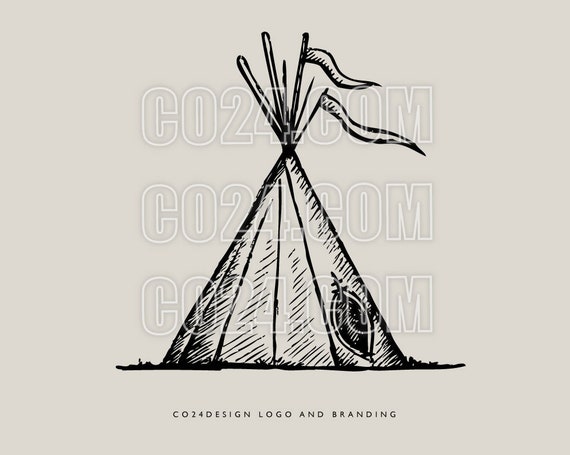This image features a black and white line drawing of a teepee on a light gray background, designed as a potential logo by CO24 Design Logo and Branding. The teepee, depicted with its poles crossing and tied at the top, has a fabric or skin draped down from approximately eight feet high. This fabric is detailed with diagonal hatch strokes to indicate shading, and an oval opening on the lower right side provides entry. The ground beneath the teepee is illustrated with small grassy tufts. At the top of the teepee, six support sticks protrude irregularly, with two on the right side adorned by pendant-shaped flags blowing to the right. The image is overlaid with three vertically stacked watermarks of the text "CO24.com" outlined in white, while below the teepee, "CO24 Design Logo and Branding" appears in smaller black font.